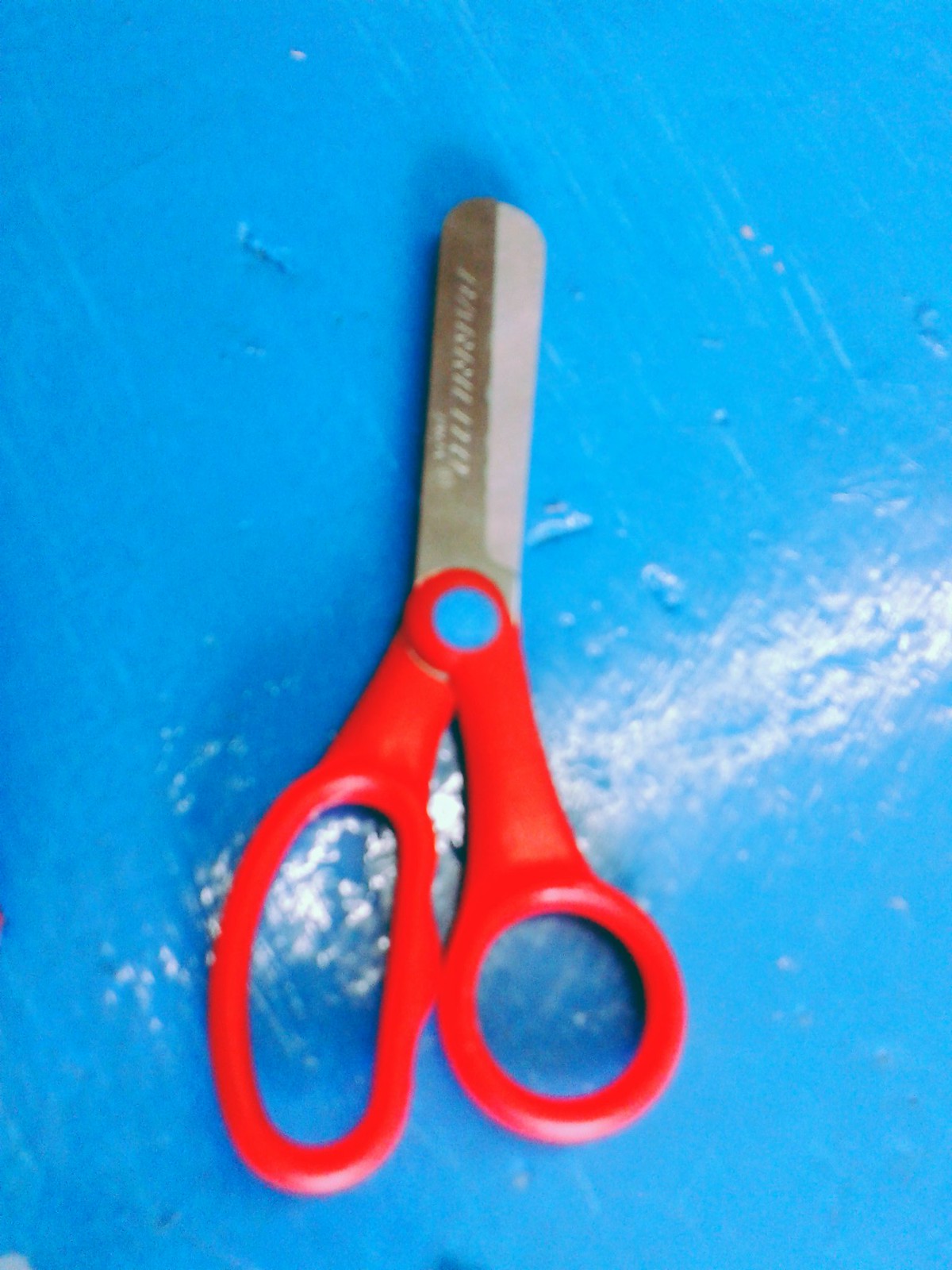The image depicts a close-up view of a pair of child’s safety scissors taken from above. The slightly vertical photograph shows the bright red handles of the scissors, positioned at the lower center of the image, with the rounded, silver-colored blades pointing upwards. The blue circular hinge connects the plastic handles to the metal blades, adding a vivid contrast. The blades have some illegible text on the bottom portion. The scissors rest vertically on a brightly painted blue surface that appears to be either a table or a floor, with visible paint streaks and dents suggesting it has been repainted. A glare from overhead lighting is present in the center of the image, enhancing the vibrant colors and indicating a likely school setting.